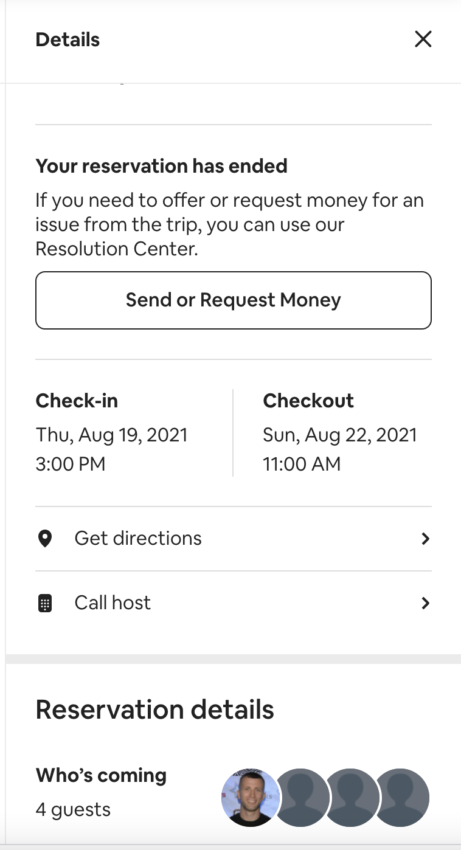**Caption:**

This screenshot from an unknown web page provides detailed information about a completed reservation. At the top, a highlighted section titled "Details" announces, "Your reservation has ended." Beneath this, users are advised to use the "Resolution Center" for any financial issues related to the trip, alongside a prominent black button labeled "Send or Request Money."

The reservation specifics are clearly stated: Check-in was on Thursday, August 19, 2021, at 3 p.m., and check-out occurred on Sunday, August 22, 2021, at 11 a.m. Additional options include "Get directions," "Call host," and "Reservation details."

A section labeled "Who's coming" reveals that four guests were part of this reservation. Adjacent to this section are four circles: the first displays a color photograph of a fair-skinned young man with short dark hair smiling at the camera, while the remaining three circles contain generic silhouettes of people.

The image's taller-than-wide aspect ratio frames all aforementioned elements, with no animals, birds, fish, plants, flowers, or trees visible in the screenshot.